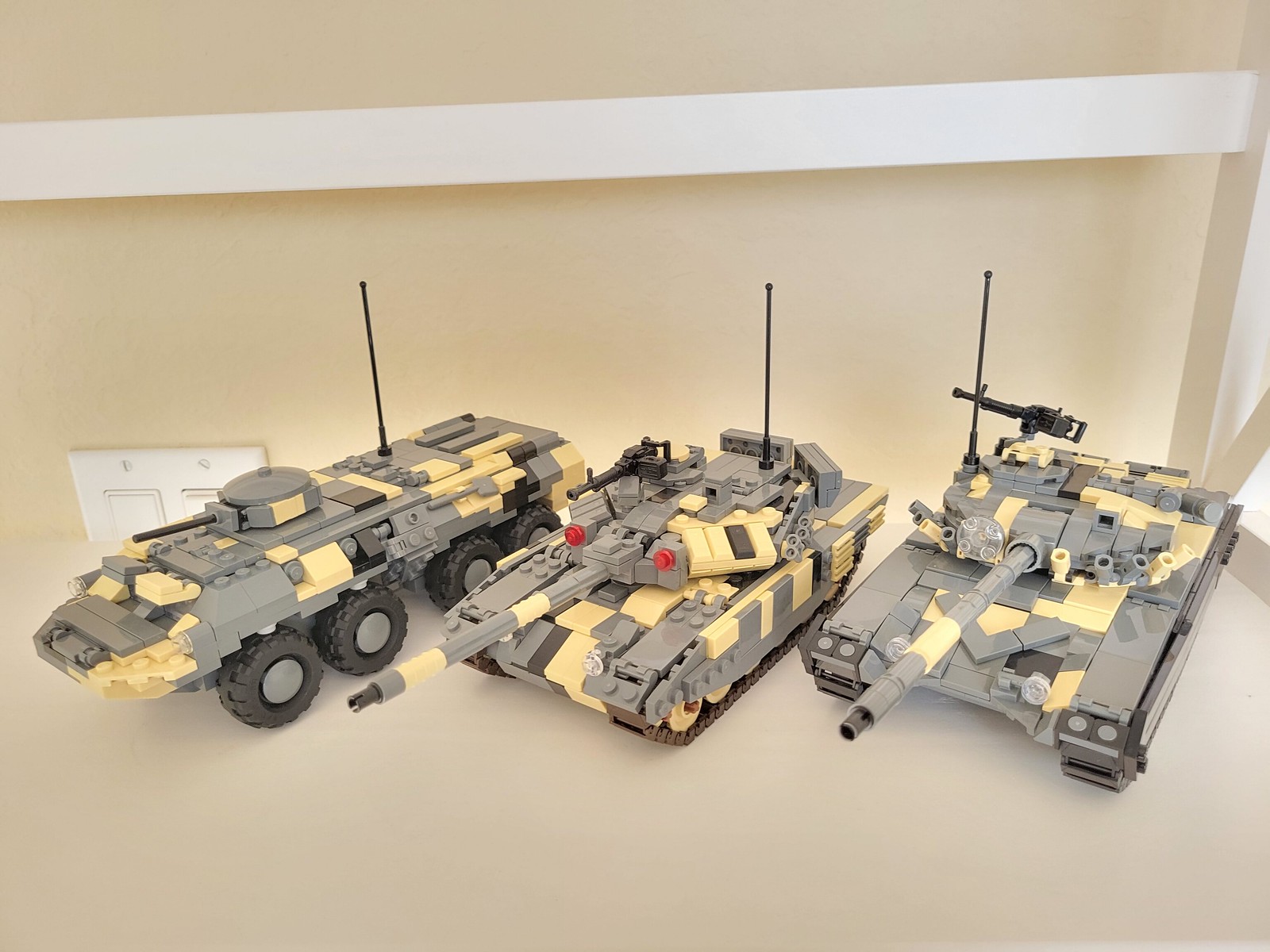This image showcases three meticulously constructed Lego models, positioned on a beige countertop against a matching beige wall, featuring white wainscoting and a nearby light switch. The two models on the right resemble traditional tanks, complete with rotating turrets equipped with cannons, machine guns, and black antennas. These tanks display a camouflage-like scheme of gray and tan bricks, interspersed with red dots and other multi-colored pieces, suggesting they might have been assembled from various Lego sets. The model on the far left, resembling a gray and yellow armored transport vehicle, differentiates itself with its eight rubber wheels instead of tank treads and a smaller turret on top. These intricate models, with their detailed construction and diverse color palette, appear to be the product of an enthusiast's careful handiwork rather than a child's simple playthings.